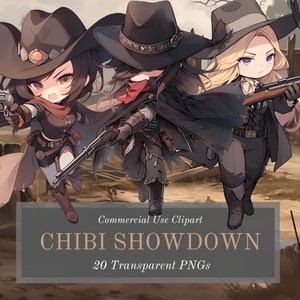This square image, rendered in a Japanese manga or anime style, features three chibi, cute female figures wearing Western-style cowboy hats and brandishing various firearms. The character on the left, with long black hair and a red scarf tied around her neck, holds a six-shooting revolver. The middle figure, whose face and hair are obscured by her bowed hat, wields a pump-action rifle and a bolt-action rifle. The character on the right, characterized by her blonde hair and blue eyes, carries a rifle as well. All three are dressed in dark brown to black jackets and boots, standing against a backdrop that suggests a sky over a dirt ground. Below the image, a text box reads: "Commercial Use Clip Art Chibi Showdown 20 Transparent PNGs."